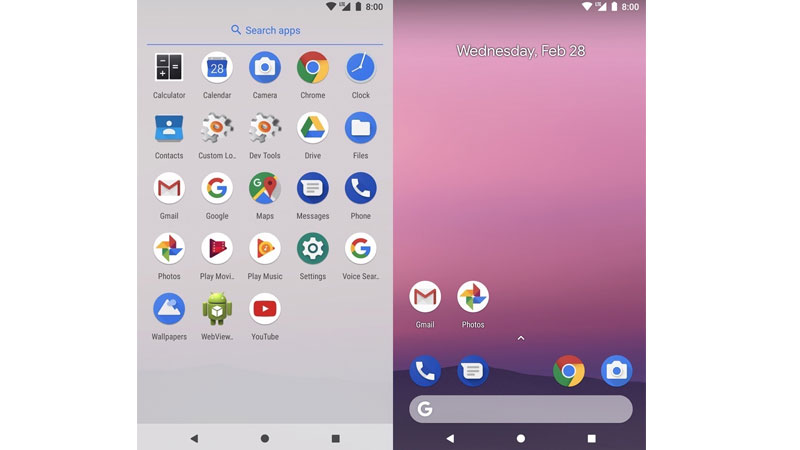The image depicts a smartphone screen with a Google-themed interface. At the very top, the status bar shows the time (8:00 AM), battery level, signal strength, and the date (Wednesday, February 28th). The main section of the screen features a "Search Apps" bar at the top, followed by a grid of app icons arranged in rows. 

The first row includes icons for Calculator, Calendar, Camera, Chrome, and Clock. The second row displays Contacts, Custom (presumably a custom app), Developer Tools, Drive, and Files. The third row contains Gmail, Google Maps, Messages, and Phone. The fourth row shows Phone (appearing again), Photos, Play Movies, Play Music, Settings, and Voice Search. Below these rows, there are additional icons for Wallpaper, Web View, and YouTube, all set against a grey background.

On the right side of the screen, there is a section with a pinkish-purple background which also displays the date and time. This area has icons for Gmail and Photos, and underneath these, there are icons for Phone, Messages, Google's search button (represented by a "G"), and Camera. Below this is a search input field marked with a "G" where users can enter information.

Overall, the interface showcases a comprehensive arrangement of apps and features housed within a visually distinct background split between grey and pinkish-purple hues.